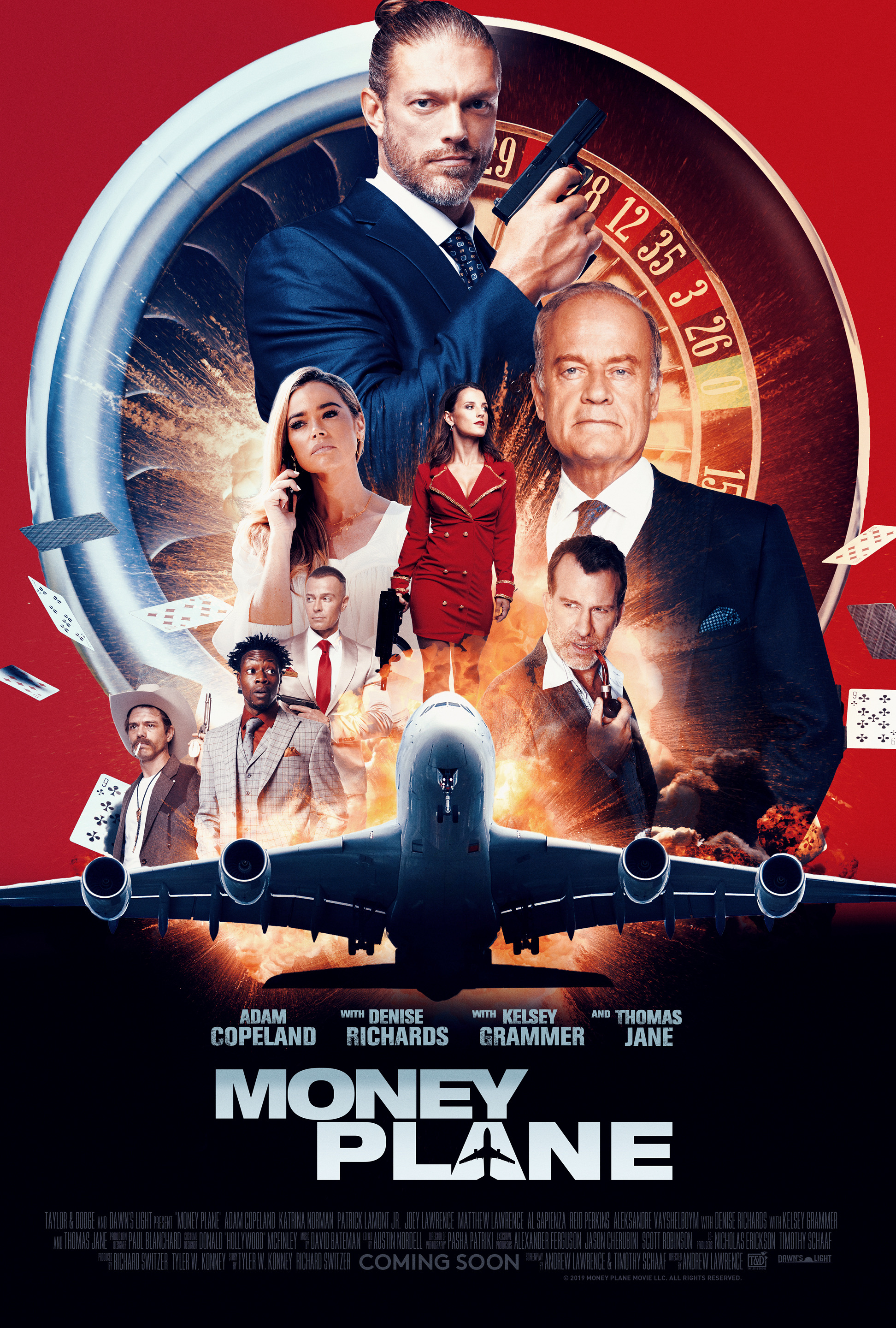This detailed movie poster for "Money Plane" features eight actors arranged in descending sizes, with the largest at the top and centering around a four-engine jet plane splitting the image. Prominently, you see Adam Copeland, Denise Richards, Kelsey Grammer, and Thomas Jane among the cast. The background blends a red roulette table and jet engine blades, symbolizing the film's high-stakes atmosphere. Cards are depicted flying in the air, enhancing the gambling theme. Kelsey Grammer, clothed in a dark jacket and tie, stands to the right as one of the larger figures. Of the two women, one is centrally located in red, while the other, slightly larger, is dressed in white. Subtle details like a cowboy figure and a character with a gun add depth to the lineup. The title "Money Plane" appears at the bottom with the 'A' in Plane cleverly designed to resemble a plane. Below this, "Coming Soon" invites viewers to anticipate the film's release. The jet's detailed exhaust and dark background complete this captivating, action-packed poster.